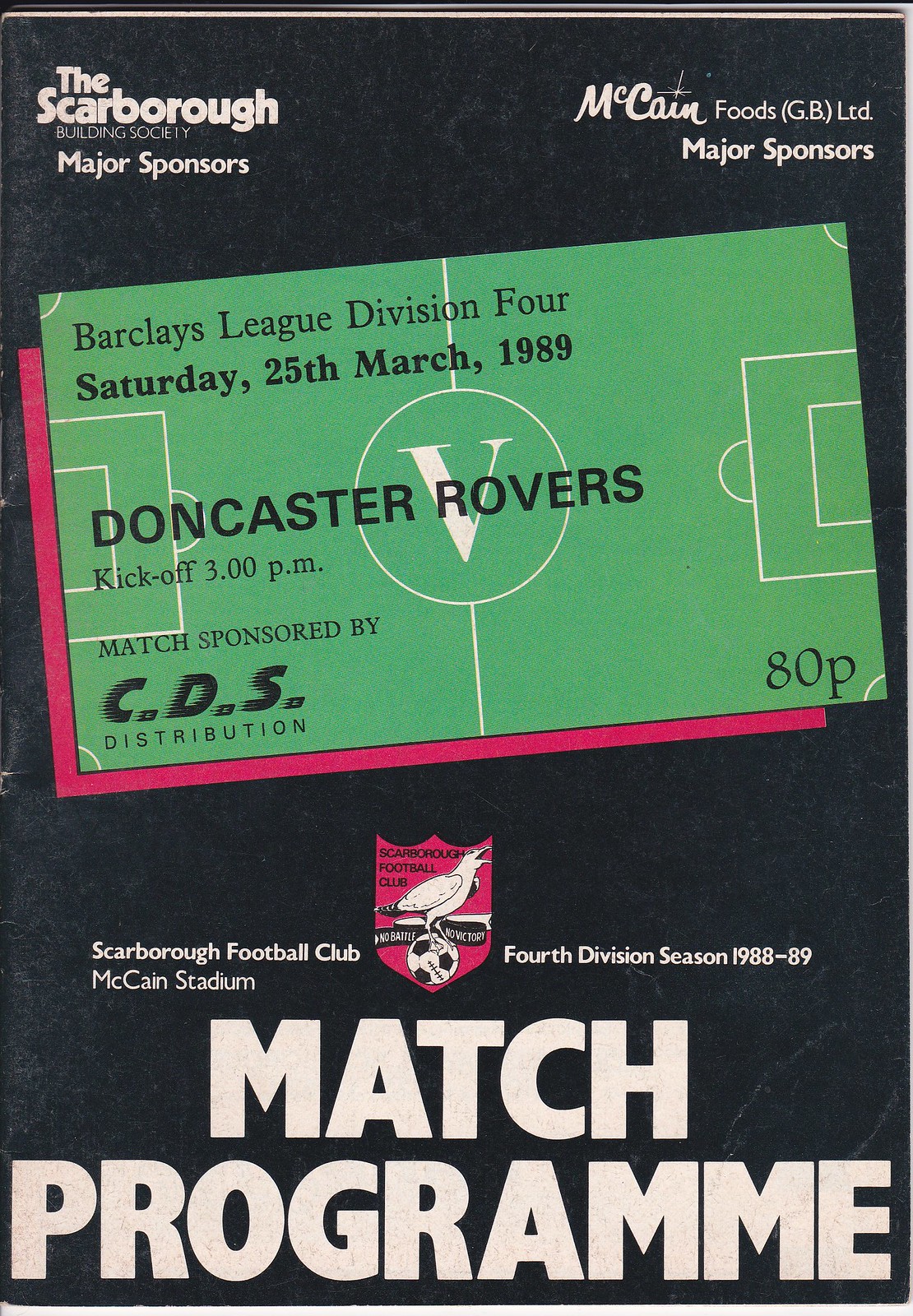This image is a tall, rectangular poster for a soccer match program, primarily black with white creases along the top and edges. The top left corner features bold white text that reads "The Scarborough Building Society Major Sponsors," while the top right corner displays "McCain Foods GBLTD Major Sponsors." Below this, a green rectangle, slanted upwards to the right, bears the layout of a soccer field with white lines, including a circle and midfield line. Black text on this green rectangle announces:

"Barclays League Division Four
Saturday 25th March 1989
Doncaster Rovers
Kickoff 3pm
Match sponsored by CDS Distribution."

Directly beneath this, to the left, lies a smaller, bright red rectangle. At the bottom of the green field, "CDS Distribution" is noted on the left and an 80 pence price on the right. A red shield with birds perched on a soccer ball appears alongside. The background of the entire layout is a black paper, with white creases along the edges, and the green rectangle's details are prominently displayed against this dark backdrop.